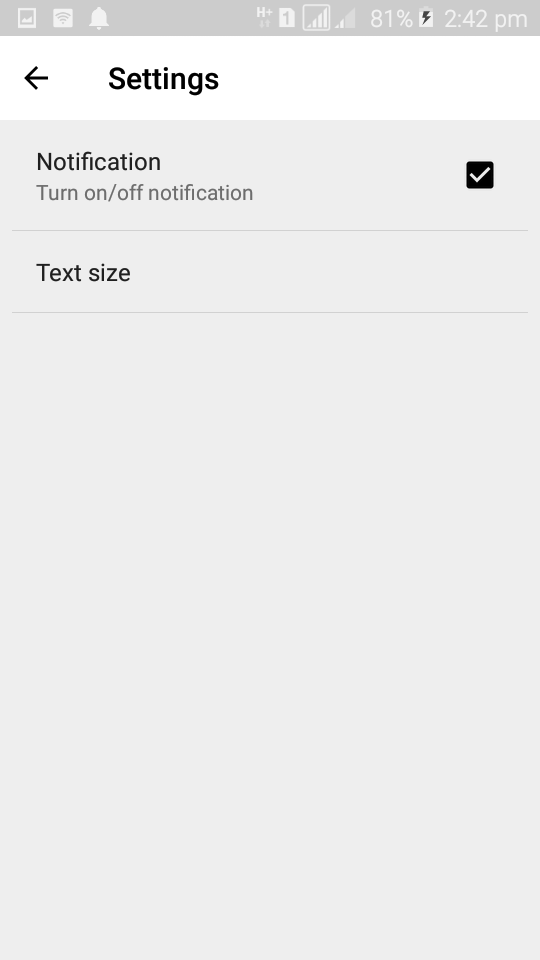In this image, which is a phone screenshot, the time displayed at the top right corner is 2:42 PM. To the left of the time, there's a battery icon with a black lightning symbol inside it, indicating the phone is currently being charged, and the battery is at 81%. Moving further left, there are two phone signal icons: the first one shows two bars out of four, and the second one shows a full four bars out of four. Adjacent to these, there's a notepad-like icon with the number one inside it, suggesting a pending notification. Additionally, there is an "H+" icon next to a numeral 11, denoting the network type and strength.

On the top left corner, there are three more icons: a photo icon, followed by a square Wi-Fi icon, and a bell icon. Dominating the top middle portion of the screen is the word "Settings" in bold black text, with a black arrow pointing left next to it. Directly below "Settings" is the word "Notification" and under that, the phrase "Turn On/Off Notification." On the far right of this line, there is a checkbox marked with a check symbol, indicating the notifications option is currently enabled.